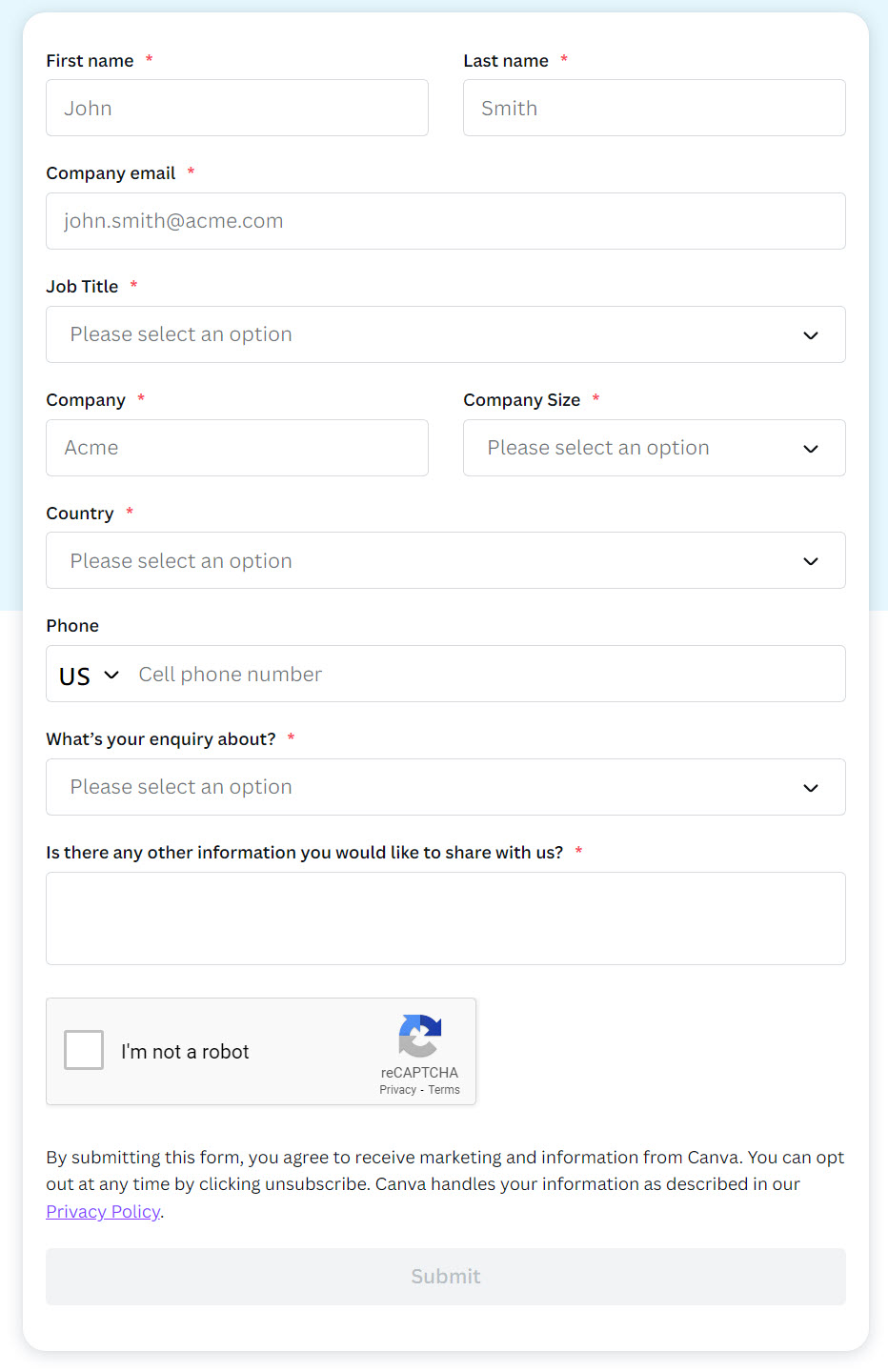The image showcases a detailed view of a form page on Canva's website designed to collect user information. The form is presented in a portrait-oriented rectangular layout. It includes mandatory fields for users to fill out, such as First Name, Last Name, Company Email, Job Title, Company, Company Size, Country, and Phone Number. The Phone Number field features a drop-down menu preset to the United States, suggesting Canva's international reach. There are also sections asking for the purpose of the inquiry—interestingly spelled with an "E"—and an open dialogue box for additional information. At the bottom, there is a "CAPTCHA" to verify the user is not a robot. The footer of the form informs users that by completing it, they consent to receive marketing communications from Canva, with an option to unsubscribe at any time. Additionally, it mentions that Canva manages user information according to its privacy policy, accessible via a clickable link.